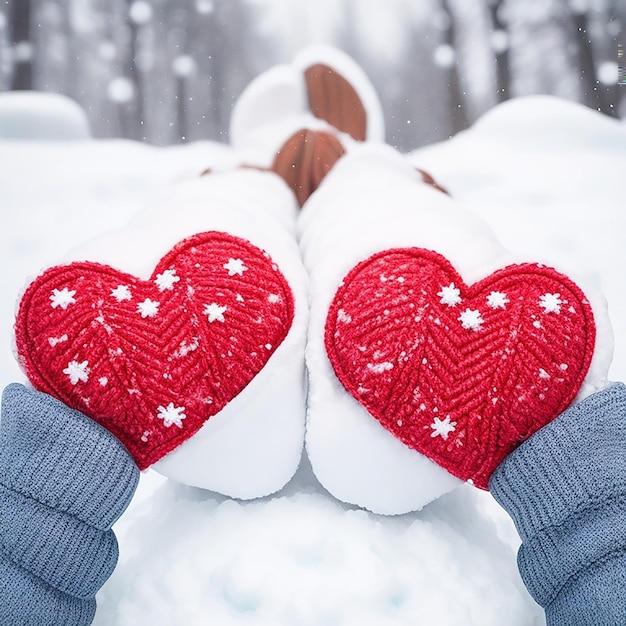A composite photograph showcases a creatively arranged scene with mostly color elements and some black and white accents. At the forefront of the image, the focus is on an imaginative placement of clothing and toys designed to resemble a figure. Strategically positioned on a white bed are the gray sleeves of a sweater, artfully angled, though notably devoid of any hands. Completing the playful ensemble are a pair of white bunny slippers adorned with hearts on the soles, adding a whimsical touch.

The upper portion of the photograph transitions into black and white, featuring softly blurred, twinkling fairy lights that enhance the dreamy and surreal quality of the composition. The meticulous arrangement and blend of color and monochrome elements create a striking and evocative visual narrative.